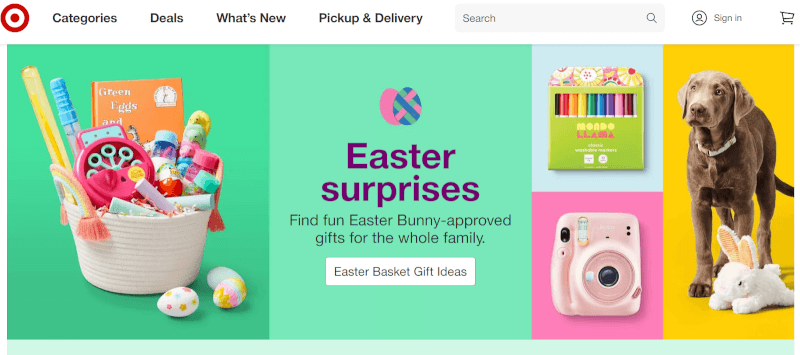This image is a Target landing page, filled with vibrant sections and a clear structure. In the upper-left corner, the recognizable Target logo, a red and white bullseye, is prominently displayed. Adjacent to the logo are several categories listed in bold gray text: "Categories," "Deals," "What's New," "Pickup & Delivery." To the right of these categories is a gray search bar bearing the placeholder text "search" in light gray, and an embedded magnifying glass icon on the right side of the bar. Further right, there's a "Sign In" option accompanied by a profile icon in gray, and a shopping cart icon indicating the e-commerce functionality.

Below this header lies a vibrant, horizontal rectangular image divided into multiple segments, each featuring colorful and engaging visuals. 

The first segment showcases a medium green background with a pink Easter basket. The basket, adorned with pink and white handles, is filled with kid-friendly items including chapsticks, foiled Easter candies, and a Dr. Seuss book titled "Green Eggs and Ham."

The second segment features a lighter green background with two overlapping colorful eggs at the top: one is solid pink, while the other is a mix of light blue, dark blue, and pink. Below the eggs, in purple text, "Easter Surprises" is written, followed by black text stating "Find fun Easter Bunny-approved gifts for the whole family." A white button underneath offers "Easter Basket Gift Ideas" in gray text.

The third segment on the right displays markers and what appears to be a pink children's camera, set on an engaging background. 

Finally, the far-right segment presents a brown short-haired dog and a plush bunny against a gold background, adding a playful touch to the overall theme.

Overall, the landing page is crafted to guide the user through various Easter-themed shopping options in a visually appealing manner.